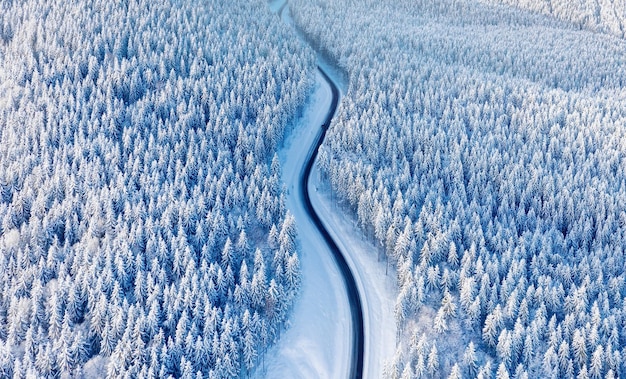In this detailed aerial photograph taken during the daytime in winter, a winding, plowed road runs through a snow-covered forest. The road, starting at the bottom center and curving slightly left and right, is framed by an expanse of pine trees adorned with white snow, creating an almost monochromatic scene despite being a full-color image. On either side of the road lies a patch of snow, and the surrounding forest is made up of dense pine trees, each blanketed in snow. The image captures the natural light of a partly sunny day, emphasizing the serene and untouched nature of this outdoor setting, with no traffic or signs of activity visible.